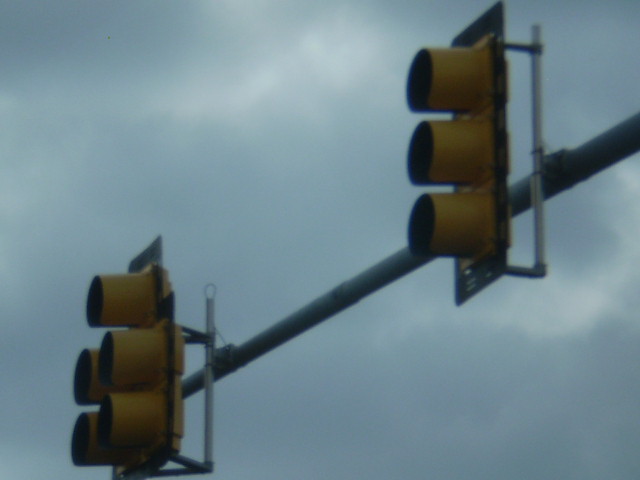This image captures a unique arrangement of traffic lights mounted on a single pole, extending diagonally from the upper right to the lower left corner of the frame. The first traffic light, positioned on the right side of the pole, features the traditional set of three circular lights, though only the yellow blinders and the black backboard are visible from this angle. To the left, there is a second traffic light configuration comprising a single light on top and a set of four additional lights arranged in two rows of two below it. Similar to the other traffic light, only the yellow blinders are visible from this perspective. The scene is set against a cloudy sky with patches of sunlight occasionally breaking through, suggesting a potentially overcast day.